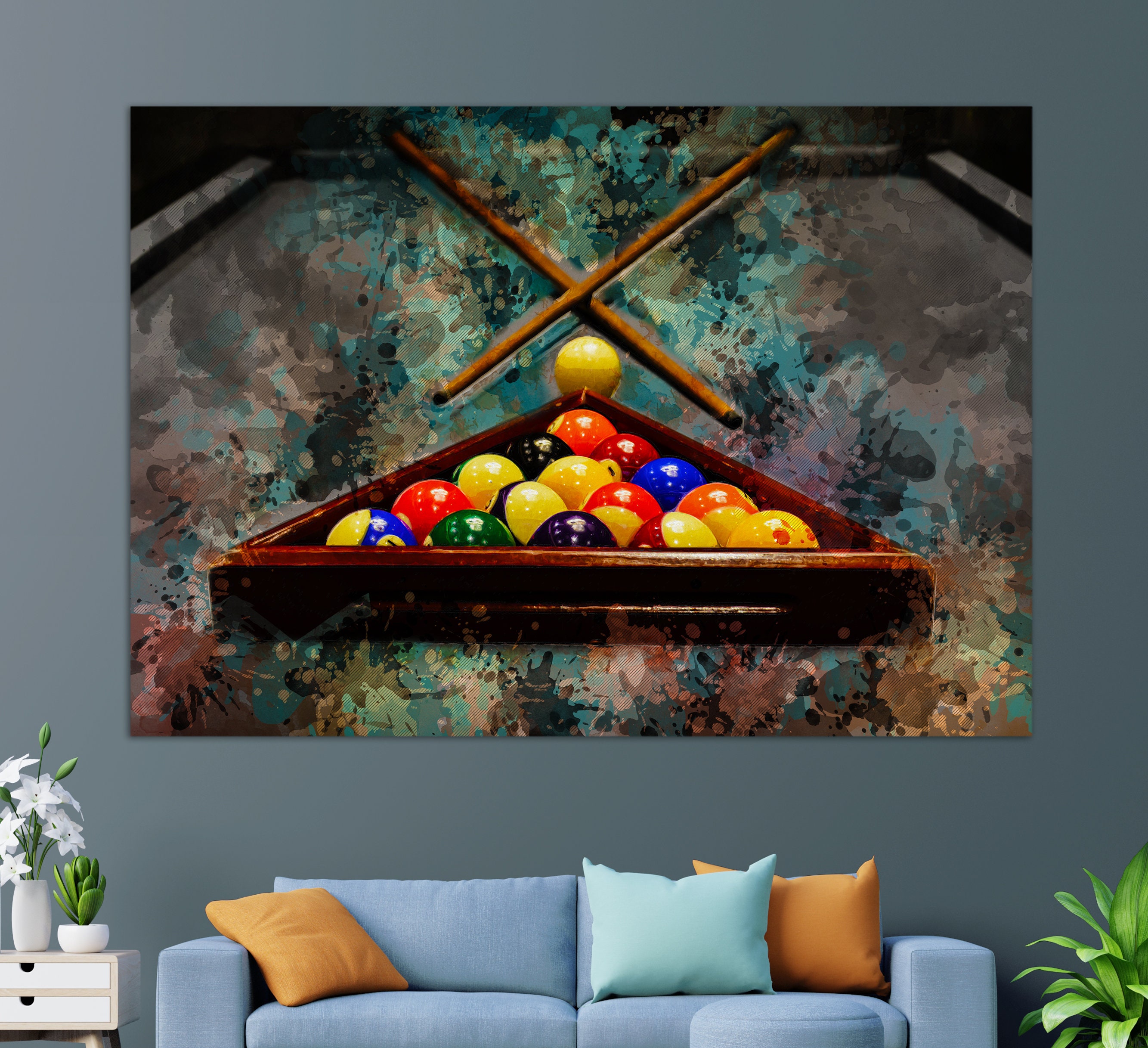The image depicts a cozy living room with a light blue couch adorned with two orange pillows and one teal pillow. Above the couch, there's a large painting featuring a close-up of racked pool balls in a triangular wooden frame, with a cue ball positioned at the tip and two crossed cue sticks above it. The pool balls display a colorful array, including yellow, orange, black, red, blue, and green hues. The background of the painting features splotches of maroon, light green, dark green, brown, peach, and purple, giving it a watercolor style appearance. 

To the left of the couch stands an off-white wooden end table with two white drawers, each having a finger-hole for easy opening. Atop the table rests a short white vase with a cactus and a taller white vase containing white flowers, with two buds still visible. On the right side of the couch is a potted plant with long green leaves placed on the floor. The wall behind everything is a green-gray color, adding a serene backdrop to the entire scene.